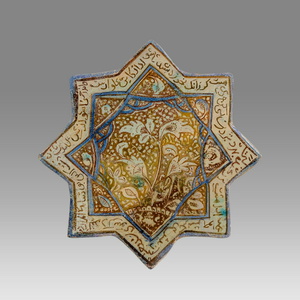The image depicts a highly intricate decorative wall piece, likely originating from India or Pakistan. The centerpiece of the artwork is an ornate eight-pointed star, which features a complex interplay of colors including gold, cream, yellow, and blue. The star is meticulously detailed, with numerous symbols or designs adorning its borders, possibly indicating text or abstract patterns. The centerpiece of the star showcases a beautiful floral motif, detailed with delicate white flowers.

The artwork is framed by two distinct blue lines, creating a layered effect that adds to its visual depth and complexity. The background transitions from a dark gray at the top to a lighter gray and finally to white towards the bottom, enhancing the prominence of the star. The star's design incorporates elements that might resemble mosaic, tile, or cork, and it is styled to give a three-dimensional appearance. The outer and inner outlines of the star form a pattern that appears to be created by two overlapping squares set at 90-degree angles, adding dynamic angles and shapes to the piece. With its rich detail and intricate patterns, the decorative piece captivates with its artistic and cultural depth, making it a striking piece of wall art.